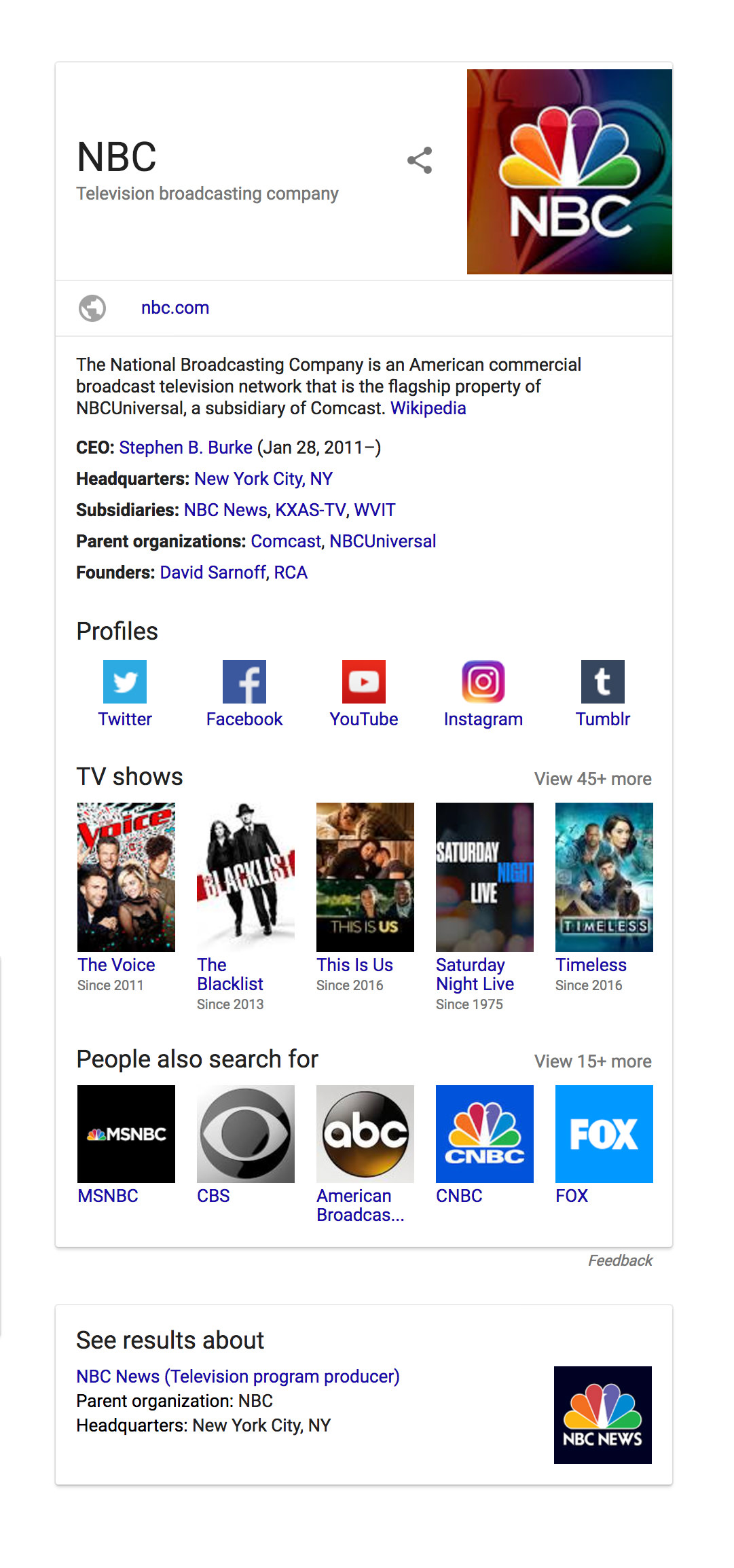![NBC Company Information Panel]

This image showcases a detailed information panel for the NBC company, reminiscent of the right-side panels typically seen on search engine results pages. The tall, white, rectangular panel features the NBC logo prominently at the top center, displaying the iconic colorful peacock feathers and the letters "NBC" beneath it. 

To the left of the logo, the text "NBC" is displayed in black, followed by "Television Broadcasting Company" in gray underneath. On the right side of the logo, there is a share link icon. Below this and encased between two thin gray lines is the website URL "NBC.com," accompanied by a small gray globe icon to its left.

The panel provides a detailed description of the company, stating in black text: "The National Broadcasting Company is an American commercial broadcast television network that is the flagship property of NBCUniversal, a subsidiary of Comcast." This description is followed by a blue "Wikipedia" link.

Further down, the panel lists several labels and corresponding details:
- **CEO:** Stephen B. Burke (in blue), with a note "(Jan 28, 2011 – )"
- **Headquarters:** New York City, New York (in blue)
- **Subsidiaries:** NBC News, KXAS-TV, WVIT (all in blue)
- **Parent Organizations:** Comcast, NBCUniversal (both in blue)
- **Founders:** David Sarnoff, RCA (both in blue)

Under the label "Profiles," icons for Twitter, Facebook, YouTube, Instagram, and Tumblr are displayed. 

The "TV Shows" section features cover photos and details for popular NBC shows, including:
- **The Voice** (since 2011)
- **The Blacklist** (since 2013)
- **This Is Us** (since 2016)
- **Saturday Night Live** (since 1975)
- **Timeless** (since 2016)

At the bottom of the panel, under "People Also Searched For," logos for other news companies are visible: MSNBC, CBS, American Broadcasting… (ellipsis), CNBC, and Fox.

A section labeled "See Results About" concludes the panel, featuring a blue link to NBC News with a description: "Television Program Producer." Below this, it’s noted in black text that NBC is the parent organization with its headquarters in New York City. The right side of this section includes the black NBC logo with the colorful peacock icon and the text "NBC News" in white beneath it.